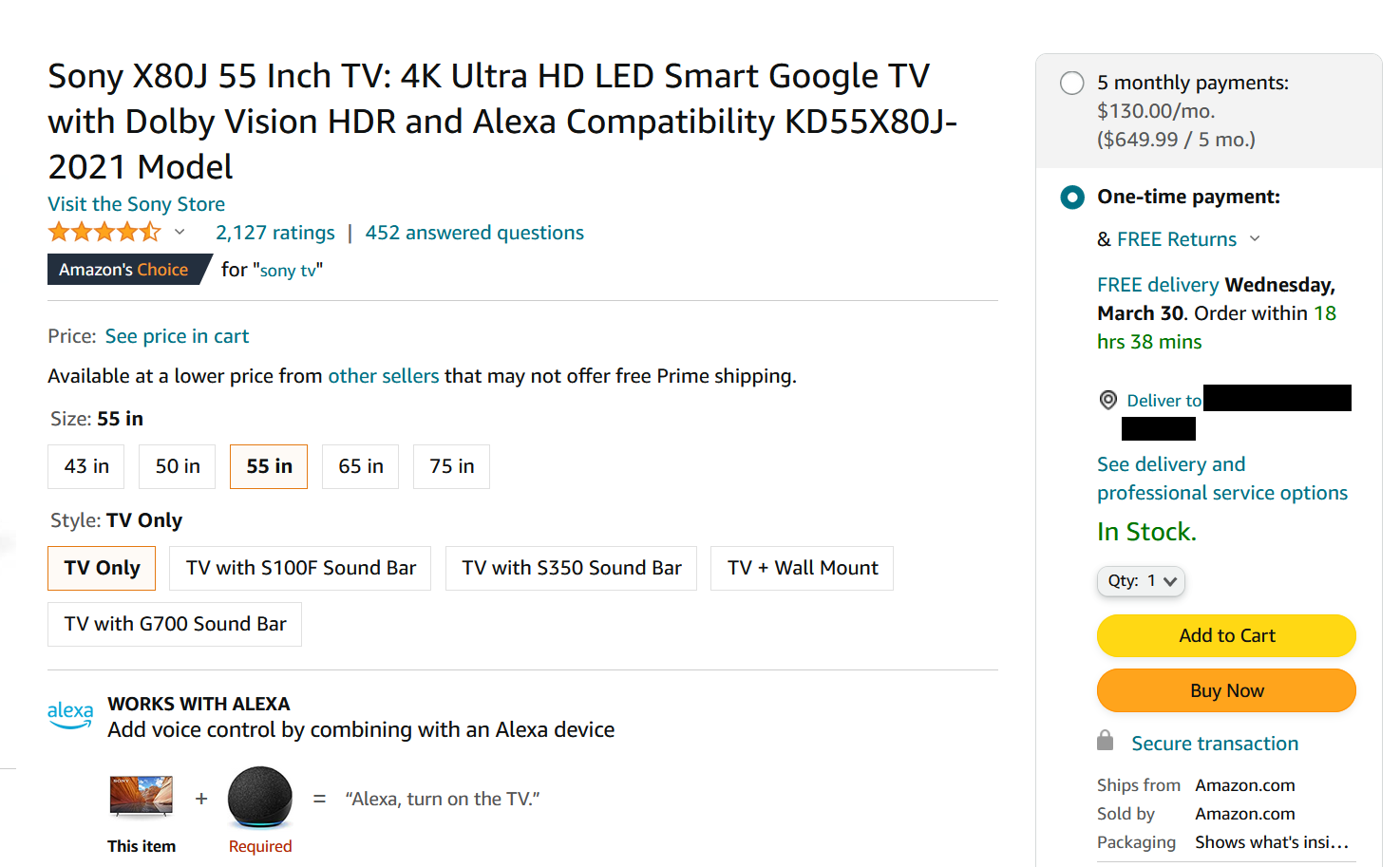The image is a screen grab of an Amazon listing for the Sony X80J 55-inch TV. Detailed at the top, the title reads: "Sony X80J 55 Inch TV: 4K Ultra HD LED Smart Google TV with Dolby Vision HDR and Alexa Compatibility," followed by specifications indicating it is a 2021 model. The page directs customers to visit the Sony store, indicated in blue text. Below, the listing showcases gold star ratings with "2,127 ratings" and "452 answered questions" highlighted in a teal shade.

The listing features an "Amazon's Choice" badge in a black and gold box, specifically for Sony TVs. The price section prompts users to "See price in cart," noting that lower prices might be available from other sellers, though such options may lack free Amazon Prime shipping.

In the product options, the selected TV size is 55 inches, highlighted in orange, with additional sizes available in 43, 50, 65, and 75 inches. The style is set to "TV Only," also encased in an orange box, while other configurations include options like "TV with Soundbar," "TV plus Wall Mount," etc.

An informational blue box indicates that the TV "Works with Alexa," encouraging users to integrate voice control using an Alexa device, illustrated by an image of the TV alongside a black Alexa device. The phrase "Alexa, turn on the TV" emphasizes this feature.

A gray box on the right side details payment options, offering five monthly payments of $130 for a total of $649.99, with the checked option being a one-time payment. Free returns and delivery by Wednesday, March 30th, are available if the order is placed within 18 hours and 38 minutes. The delivery section also mentions professional service options, with delivery details obscured for privacy.

A black icon pin and a "Deliver to" line lead to a summary indicating the item is in stock, to be added to the cart using the gold "Add to Cart" or "Buy Now" buttons. A gray padlock symbol denotes a secure transaction, clarifying that the item ships from and is sold by Amazon.com. Packaging options are provided, with an option to reveal what's inside.